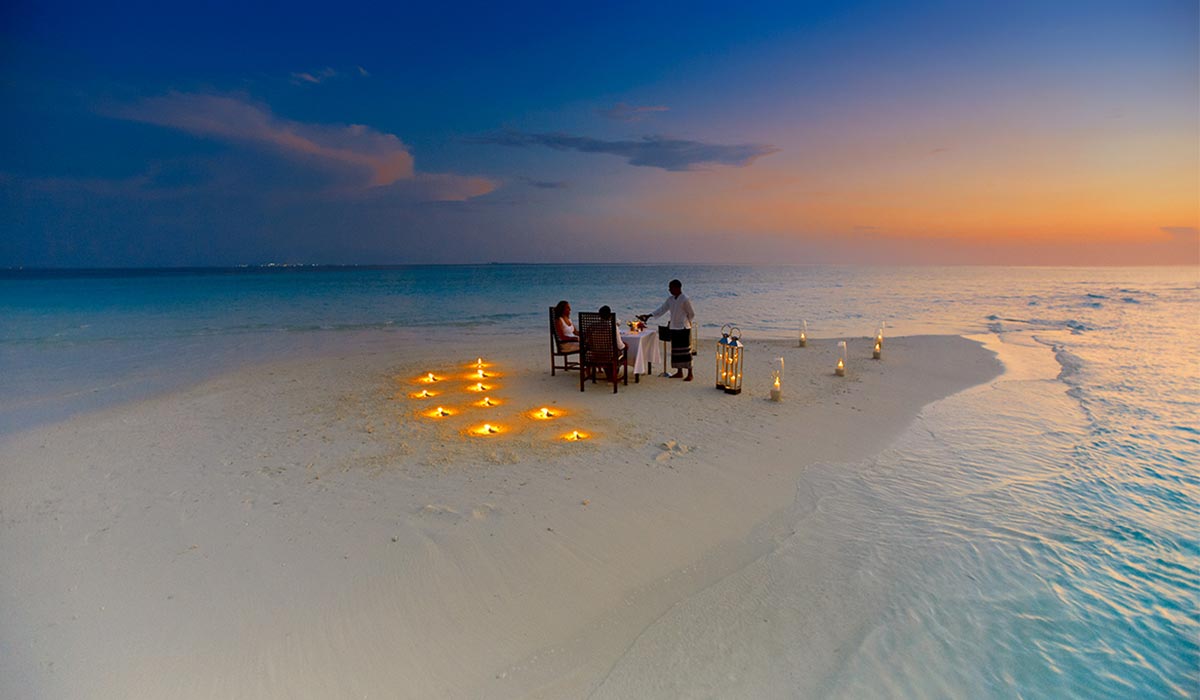This serene photograph captures a romantic candlelight dinner set on a pristine white sandy beach during low tide, where the sand is still visible around both sides of the scene. The setting sun casts a breathtaking array of blue, pink, and yellow hues across the sky, creating a stunning backdrop to the evening. Centered in the photo are two individuals seated at a white-clothed table adorned with soft orange lanterns, contributing to the ethereal ambiance. They sit in high-back wooden chairs dressed in white, exuding elegance. Serving them is a waiter, also dressed in white, enhancing the scene's tranquil, spiritual atmosphere. The expansive ocean with its calm, light blue waters adds to the overall serenity and beauty of this intimate beachside dinner.